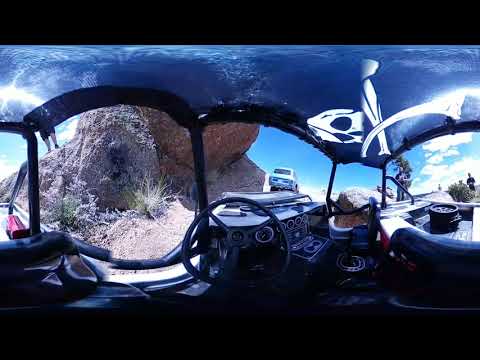This photograph appears to be taken from within an off-road vehicle, possibly a panoramic shot that has caused some warping of the steering wheel, giving it a deformed circular shape. The vehicle itself seems rugged, lacking window panes but equipped with a roof, indicating its design for outdoor and potentially rough terrains. The setting is bathed in bright sunlight, likely midday, under clear blue skies, suggesting a warm, possibly desert-like environment with hints of green growth.

In front of the vehicle, there’s an old coupe, potentially another off-road vehicle, seemingly souped-up for the terrain. The landscape includes a prominent large rock directly ahead of the steering wheel, strengthening the impression that the vehicle is actively navigating a rocky, mountainous path.

The scene is framed by a black border at the top and bottom, and the photo features a wide array of colors including blue, white, gray, brown, tan, black, red, green, and pink. There are also reflections and light patterns that create the illusion of being underwater, although it is clear that the setting is terrestrial. A white symbol bordered in dark lines appears near the top right of the image. No text is present, and no people are visible, although one mention of a silhouette might suggest a vague human figure on the right. The overall interior perspective is dark blue, with light and shadows adding to the complex visual textures.